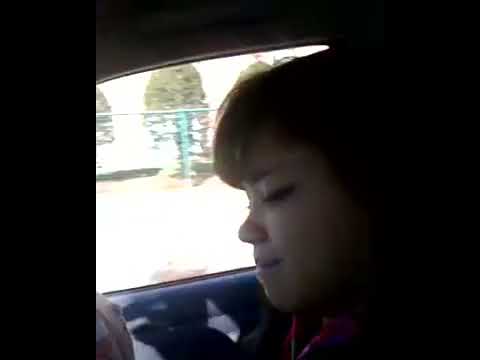The photograph captures a side profile of a young teenage girl, possibly with brunette or black hair, sitting in the passenger seat of a car. Her head is turned to the left, eyes closed or looking down, and she appears to be subtly grinning. The lighting casts a shadow over much of her hair, making it difficult to determine its exact color or length. The background outside the car window features a blurry, sunlit scene with grass, trees, and a faintly visible fence. The image is vertically cropped with black bars on either side, enhancing the focus on the girl at the center. The car door and some dark blue fabric are visible in the periphery, adding context to the scene. The overall atmosphere suggests a peaceful, reflective moment as she gazes downward, perhaps at a phone or simply lost in thought.